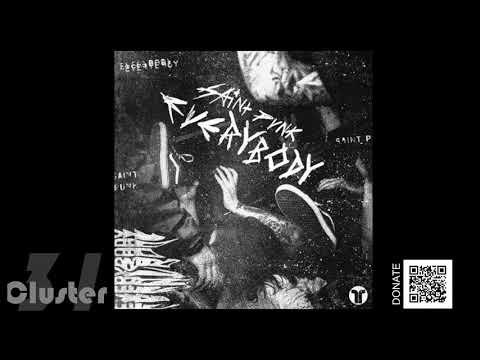This image, appearing in black and white, seems to be a poster or album cover. The background is solid black, framing a central square image where a chaotic blend of intertwined bodies is depicted. Visible are several sneakers, arms with hands, and the backs of human heads. 

Prominently, bold white text across the center reads, "Saint Punk Everybody," with stylized, angled lettering. The scene captures a dense, almost tumultuous grouping, possibly portraying a dynamic crowd or mosh pit. Detailed within the entanglement, you can notice a tattooed arm and multiple legs, suggesting the entwined bodies of different individuals. 

In the lower corners of the image, additional elements lend further context: the bottom left corner features the word "Cluster" alongside a large numeral "3" partially obscured behind it, while the bottom right corner displays a QR code with the word "DONATE" written vertically in all capital letters beside it.